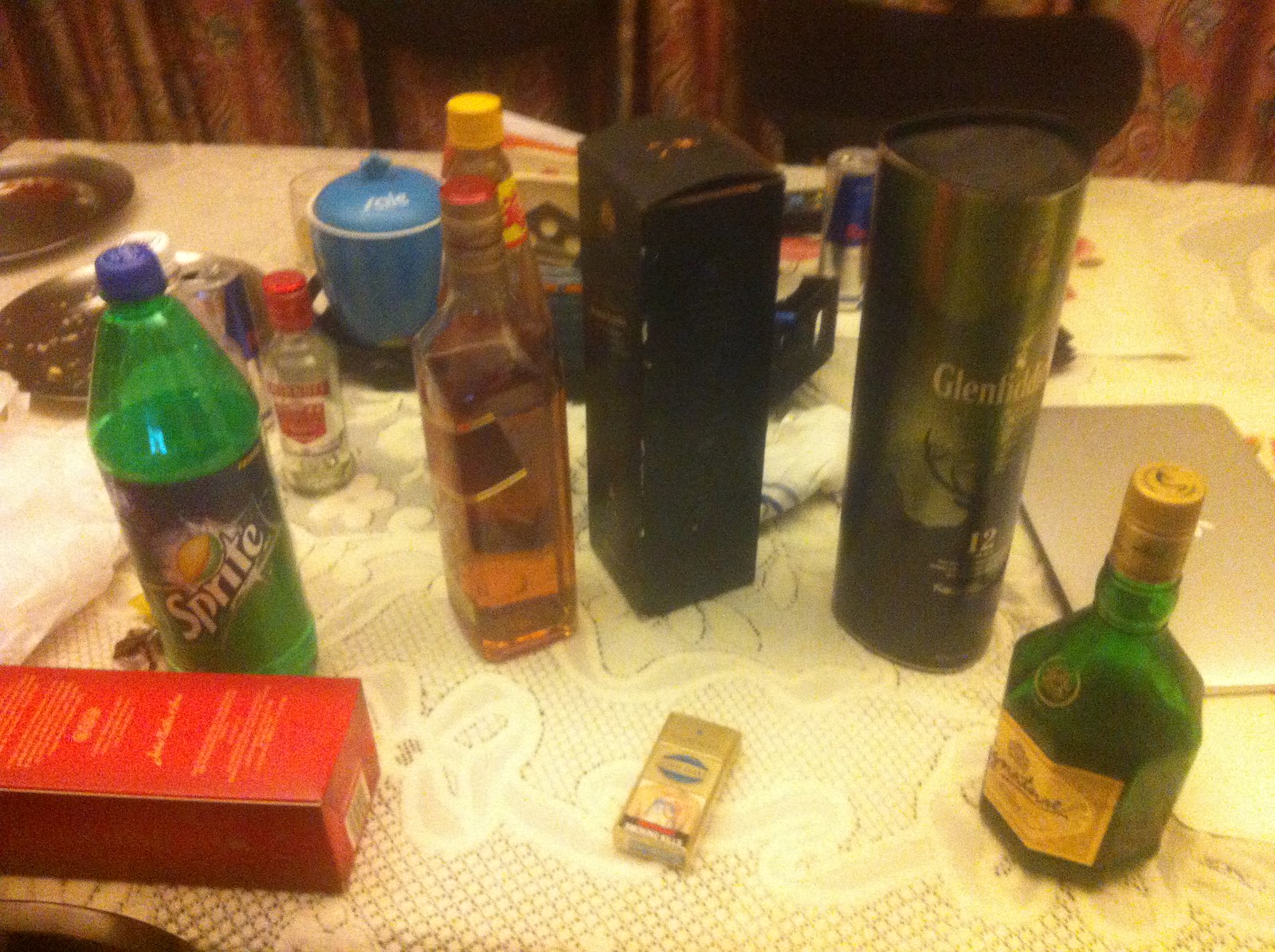The image depicts a cluttered table covered with a white tablecloth overlain by a lacy one, viewed from a slightly top-down, diagonal perspective. On the left is a green bottle of Sprite with a blue cap, featuring the classic Sprite logo with lemon and lime imagery. Adjacent is a bottle of booze, partially obscuring a bottle of hot sauce. A black tall cardboard box with gold writing, most likely another alcoholic beverage, is situated about an inch to the right. Further right, around two-thirds across the image, is a cylindrical black container labeled "GLEN" with the remaining text obscured by glare and adorned with a deer emblem, indicating a Glenfiddich whiskey. In the lower right corner sits another green bottle with gold accents. The table also holds smaller bottles, cans, a pack of cigarettes, two silver serving trays on the top left, and a red box and blue-lidded jar toward the back. Additionally, a laptop and the tops of two brown chairs are visible in the background. The scene is set against a backdrop of reddish-brown, gold, and green paisley curtains hanging at the top of the image.